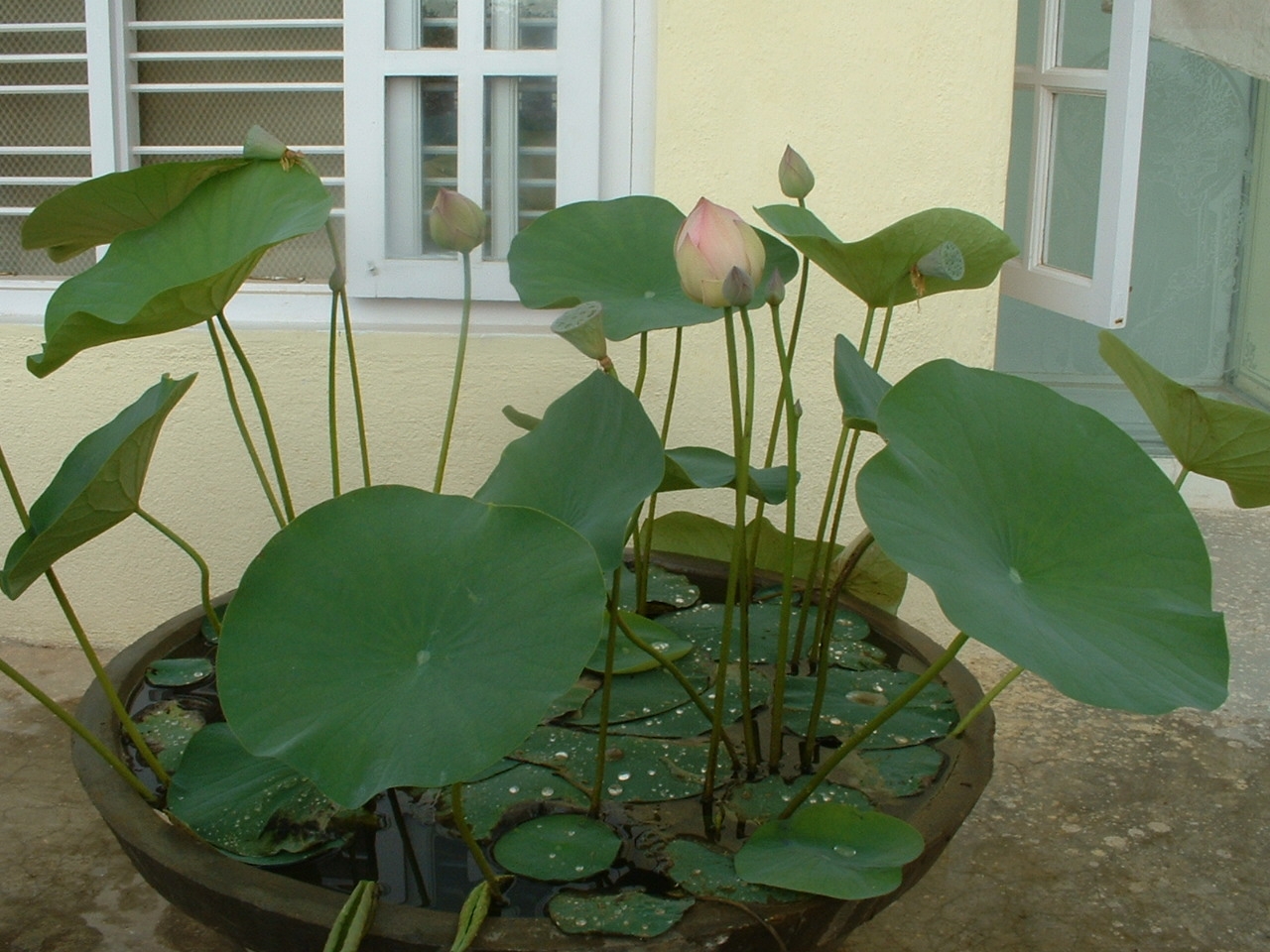In the foreground of this image, a large dark brown flower pot sits prominently at the bottom center, filled with water and adorned with green lily pads and flowers, some of which have pink blooms at the end of long stems. The surface surrounding the pot appears to be a concrete walkway, indicative of an outdoor setting. Moving upwards within the image, the background reveals a light yellow house with white-trimmed rectangular windows. One window, positioned towards the upper left corner, has bars across it and partially obscured glass, suggesting the presence of shades or blackout curtains behind it. To the upper right of the image, a door is visible. The overall scene is bright and clearly illuminated by natural daylight, emphasizing the midday timing. The colors in the image range from the whites and yellows of the building to various shades of green, pink, brown, gray, and black, lending a vivid and detailed depiction of the outdoor area in front of someone's home. There is no visible text anywhere in the image, making the focus purely on the physical details and setting.